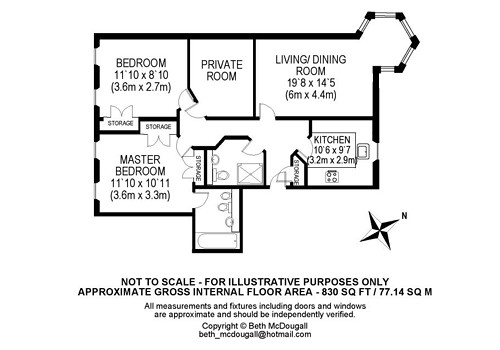The image is a detailed floor plan of a house depicted in a rectangular landscape orientation, featuring a unique pentagon-shaped corner and a small protruding section at the lower part identified as a bathroom. Below the floor plan, a disclaimer reads: "Not to scale. For illustrative purposes only. Approximate gross internal floor area 830 square feet (77.14 square meters). All measurements and fixtures, including doors and windows, should be independently verified." The copyright information is attributed to Beth McDougall (beth_mcdougall@hotmail.com).

In the bottom right corner, there is a compass indicating the orientation with 'N' pointing towards the top-right corner. The layout includes various labeled rooms: a bedroom, a master bedroom, a kitchen, a living/dining room, a private room, and storage areas. Some spaces resembling bathrooms are present but unlabeled. Each room’s dimensions are provided in both feet and meters.

The pentagon-shaped section appears to be an additional space, possibly a solarium or conservatory. The floor plan indicates windows and doors with black outlines. Overall, the plan offers an aerial view of the house layout, emphasizing the spatial arrangement and dimensions of each room.